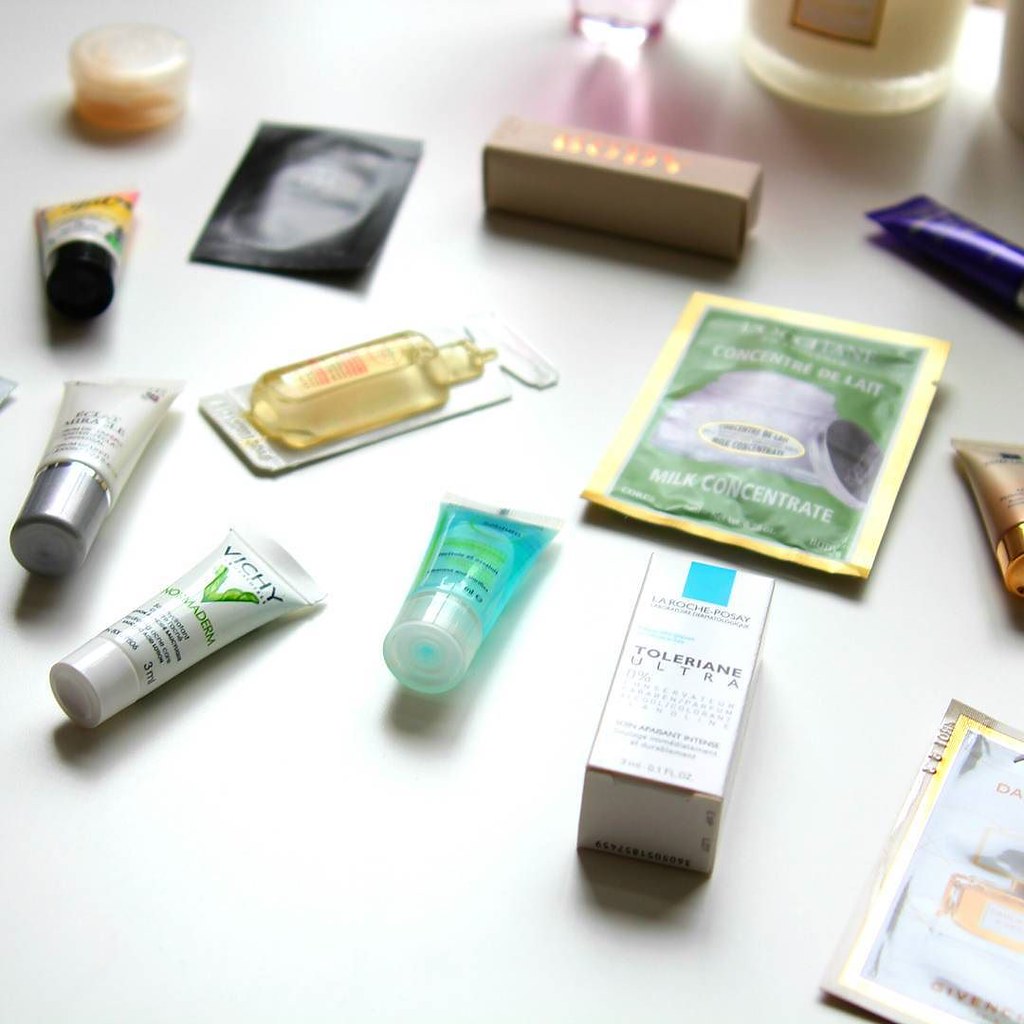This image, slightly taller than it is wide, features a well-organized display set against an off-white countertop. The layout carefully spaces each item an inch or two apart, enhancing clarity. The arrangement begins about 20-30% up from the lower left corner, leaving that section empty.

1. **Vichy Tube**: A small, off-white tube labeled "Vichy" with a V-shaped leaf logo.
2. **Aquamarine Gel Tube**: Positioned to the right of the Vichy tube, this small, clear gel is aquamarine in color.
3. **Toleriane Ultra Box**: Another small box, labeled "T-O-L-E-R-I-A-N-E Ultra", lies to the right of the gel tube.
4. **Partially Visible Item**: In the lower right corner, an item with a light blue and white background, framed by a yellow border, is partially cut off.
5. **Gold Tube**: Directly above the partially visible item.
6. **Green Packet**: Positioned above the gold tube, featuring a yellow outline and labeled with "milk concentrate" at the bottom.
7. **Air Freshener Insert**: This item, resembling a plug-in air freshener insert, is to the left of the green packet.
8. **Off-White Tube with Silver Cap**: Directly to the left of the air freshener insert.
9. **Additional Tubes**: Behind the off-white tube are at least four similar items.

The composition of this image showcases a variety of personal care products, neatly arranged for visual appeal.